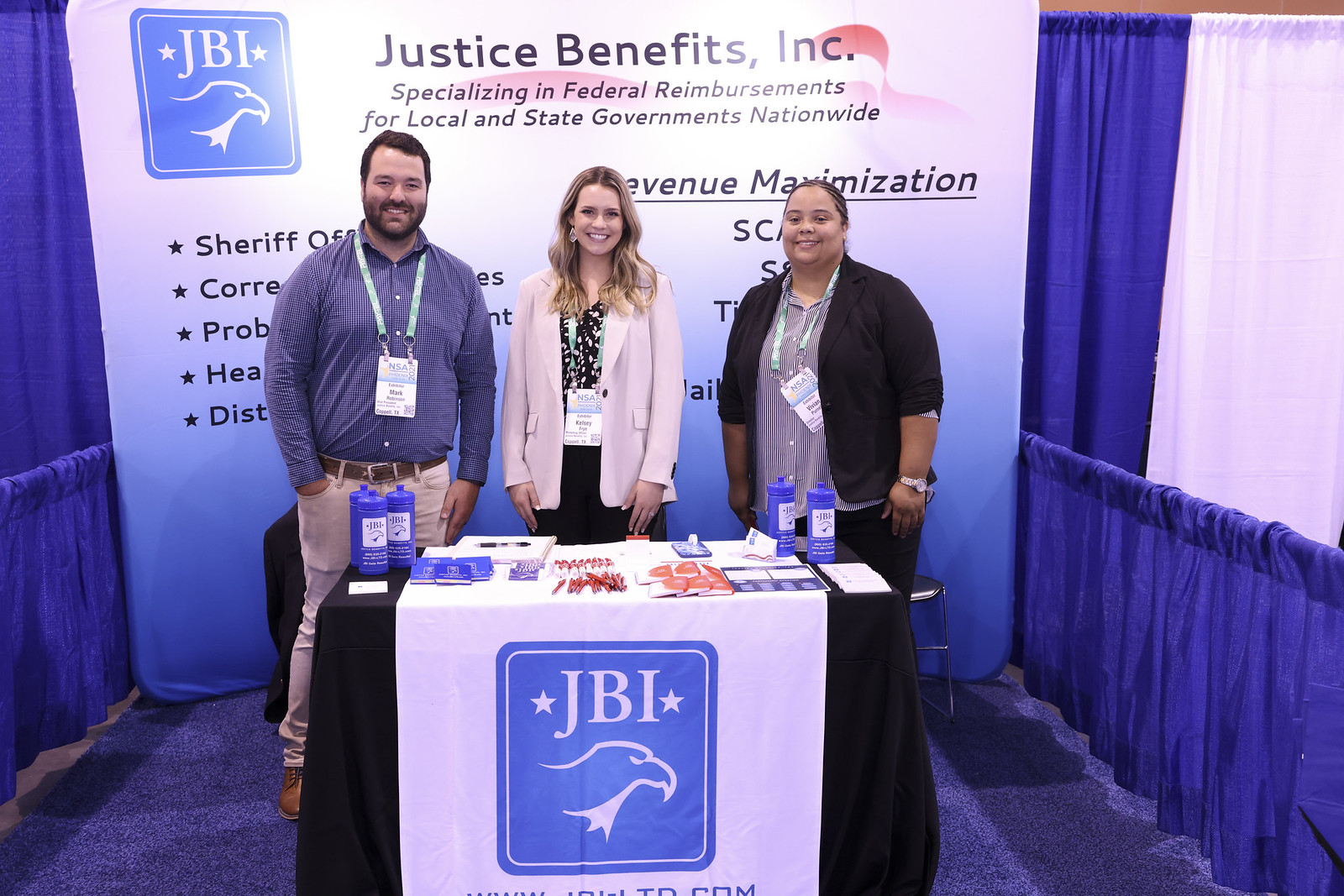In a bustling convention setting, a photograph captures a booth manned by three individuals— a man on the left and two women in the middle and right positions. The table before them is adorned with a black tablecloth featuring a pronounced white stripe down the center, drawing attention to a blue box prominently displaying the letters "JBI" in white with an eagle’s head outline. The tabletop is scattered with an array of promotional materials including pamphlets, pens, and blue water bottles, all branded with the JBI logo.

Behind the trio stands a large white billboard, conspicuously marked with the JBI symbol on the top left and the text, "Justice Benefits Incorporated specializing in federal reimbursements for local and state governments nationwide," in bold black font on the right. The backdrop for this scene includes dark blue curtains and a smaller segment of white curtain on the right, complemented by waist-high dividers draped in blue fabric. 

Each person behind the table is distinctly dressed: the man on the left sports a blue plaid shirt paired with white khaki pants and a leather belt, exuding a casual yet professional look. The woman in the middle, with cascading long wavy blonde hair, stands out in a pink suit coat over a black-and-white spotted shirt and black pants. To the right, a brown-skinned woman has her hair neatly tied back, wearing a sharp black suit coat over a blue and white striped shirt, and black pants, exuding a polished and formal demeanor. The carpeted floor and the detailed setup of the booth contribute to the organized and professional atmosphere, indicative of the convention's formal environment.